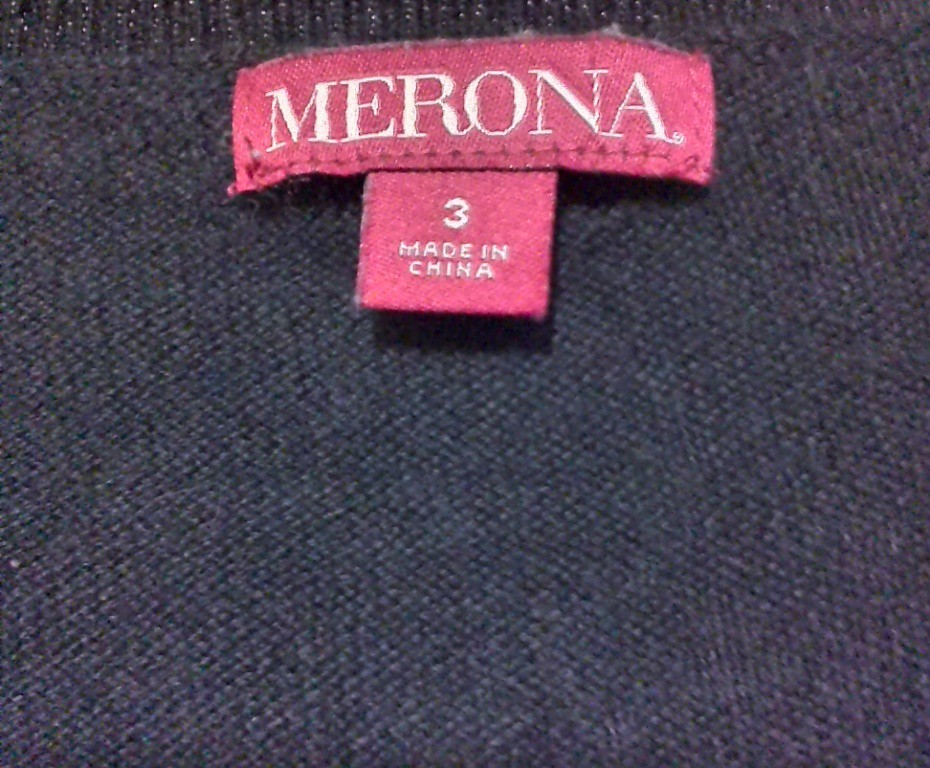This photograph captures an extreme close-up of a sweater's neck tag. The entire background consists of the dark gray-blue fabric of the sweater, highlighting its texture. Dominating the frame is a magenta neck tag with crisp white font bearing the brand name "MERONA," complete with a small trademark symbol nestled at the base of the final "A". Just below this brand tag, a smaller, square-shaped magenta tag is visible, featuring a white number "3" and the text "Made in China." The fabric of the sweater appears somewhat translucent, subtly revealing a white background layer underneath.